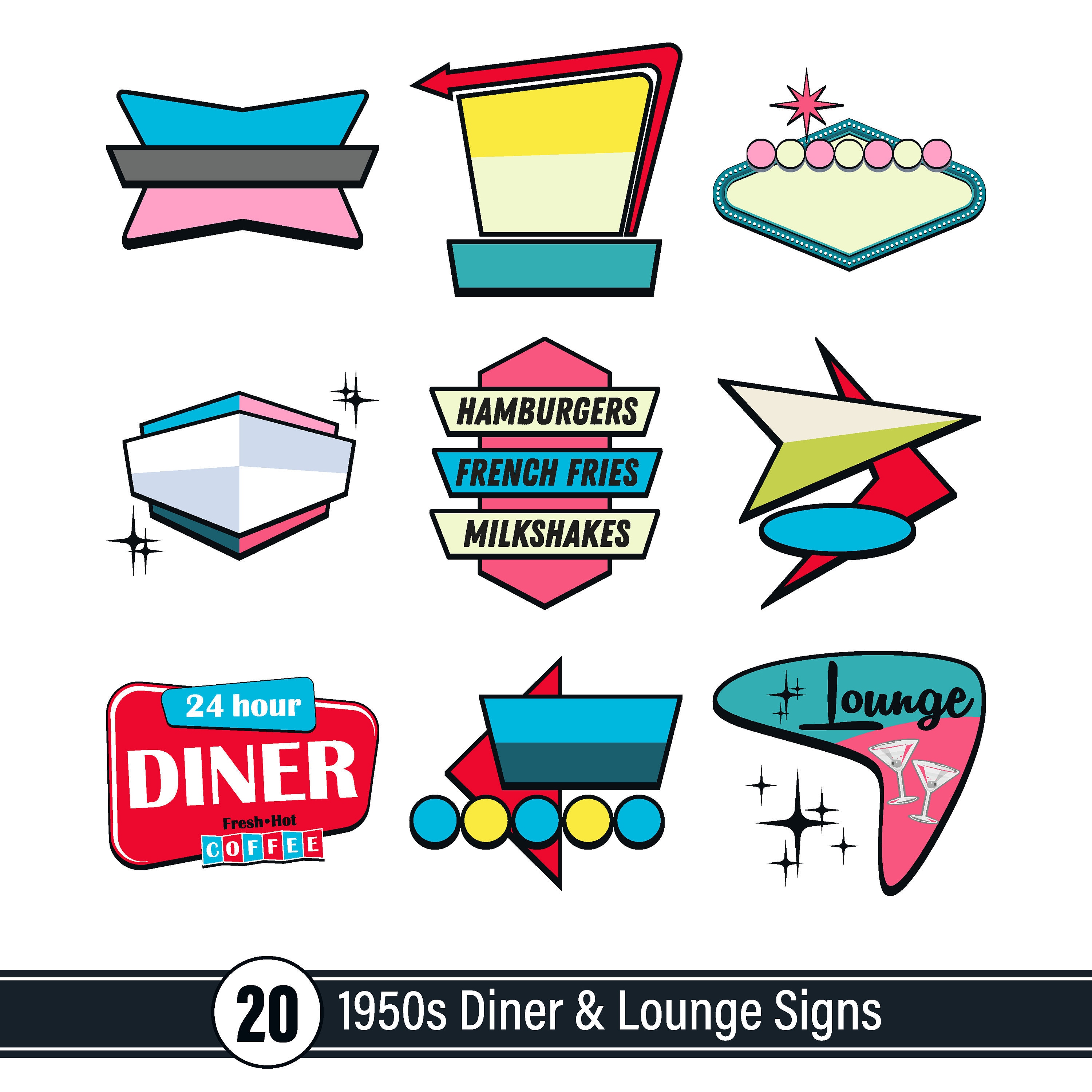This image is an infographic showcasing nine computer-generated, cartoon-style renderings of various 1950s diner and lounge signs against a white background. At the bottom of the image, a gray stripe contains white text reading "20 1950s Diner and Lounge Signs," and includes a circular logo with black "20" on a white background.

From top to bottom, left to right, the signs include: 

1. A blue and pink star-shaped sign.
2. A yellow square circle with a red arrow overlay.
3. A round sign resembling the Las Vegas sign, adorned with a star at the top and pink and yellow circles.
4. A pink and blue squared sign.
5. A red, yellow, and blue sign in the middle displaying "Hamburgers, French Fries, Milkshake."
6. A yellow arrowhead pointing at a red arrow.
7. A red and blue "24-Hour Diner" sign featuring additional text, "Fresh Hot Coffee," in alternating blue and red blocks with white lettering.
8. A geometric shape, consisting of a red and yellow trapezoid on top of a triangle.
9. A light blue and pink "Lounge" sign adorned with two martini glasses.

The overall design captures the vibrant and varied aesthetic typical of 1950s diners and lounges.